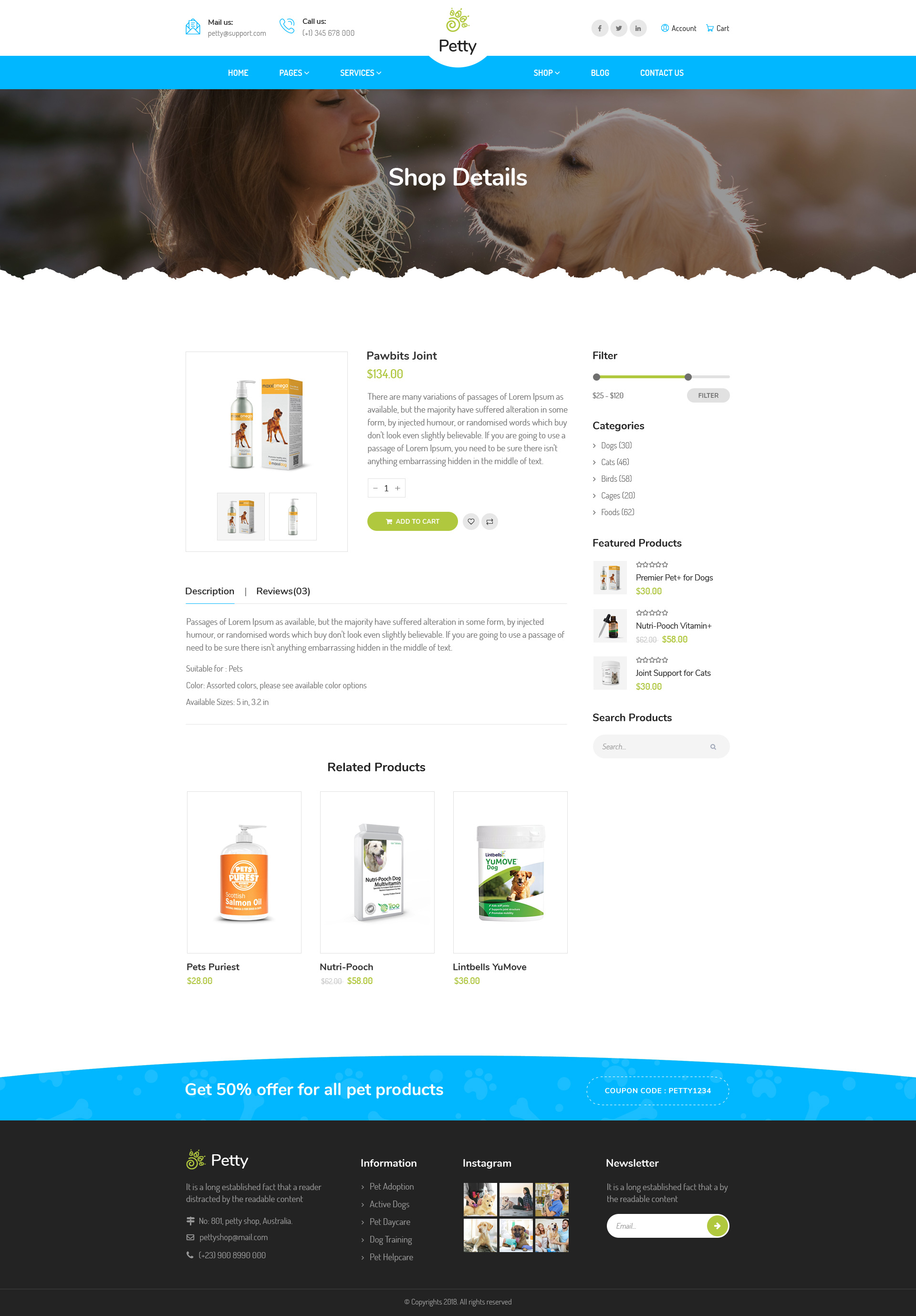In a vibrant and engaging scene, there's a woman smiling warmly as she looks down at her dog, which is adorably licking its nose. The visual conveys the joyful bond between the two. Adjacent to this heartwarming interaction, various elements of the digital interface can be seen, suggesting an online pet supply store.

The top part of the screen features tabs for "Home," "Services," "Shop," "Blog," "Contact Us," and "Shop Details." Additionally, links to social media platforms like Twitter and LinkedIn are present, indicating active engagement on those fronts.

A promotional banner highlights the product "Premier Pet Plus for Dogs," boasting joint support vitamins available for $134. This section emphasizes a variety of pet products, ranging from food and supplements to cages and accessories for cats, dogs, and birds. The advertisement suggests the products are high-quality with a touch of humor, though it recommends carefully reviewing text details to ensure accuracy.

For a limited time, a coupon code "PETTY1234" is prominently displayed, offering discounts on all pet products, suggesting a user-friendly and appealing shopping experience.